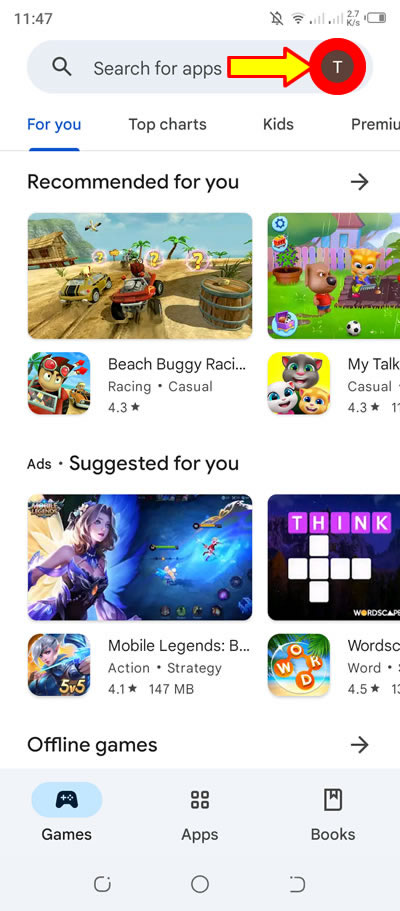This vertically rectangular screenshot from a cell phone displays a predominantly white background. At the top left corner, the time reads 11:47, while the top right corner shows several status icons, including the alarm (off), Wi-Fi signal bar, and battery level. Beneath these indicators is a search bar for apps featuring an overlaid large yellow arrow with a red border pointing from left to right. This arrow directs attention to a "T" inside a black background, encircled by a large red ring.

Directly below the search bar is a horizontal menu featuring options such as View, Top Charts, Kids, and Premium. Underneath this menu is a section titled "Recommended for you," displaying icons for two game apps side by side; however, the game on the right is cut off, while the visible game is "Beach Buggy Racing."

Further down is a section labeled "Ads suggested for you," featuring two more game icons side by side, with the right game icon also cut off. The visible game is "Mobile Legends: Action Strategy," rated at 4.1 stars. A suggestion for "Offline Games" follows, accompanied by an arrow icon. Finally, at the very bottom of the screenshot, we find selection icons for Games, Apps, and Books.